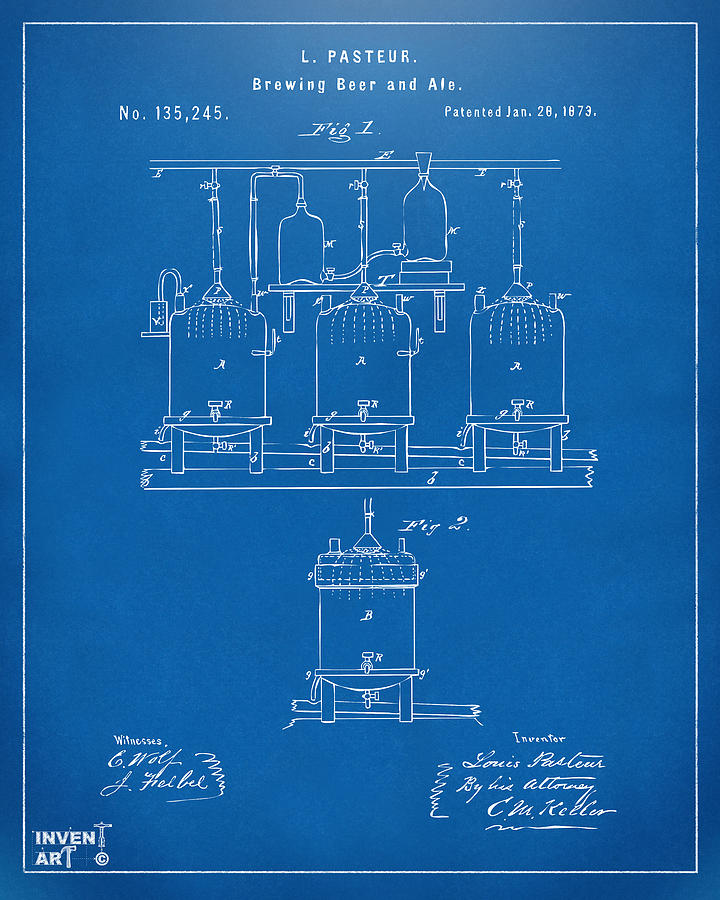The image is a detailed blueprint-like diagram with a blue background and white text and illustrations. At the top, it reads "L. Pasteur, Brewing Beer and Ale, Number 135245, Patented January 28, 1873." Below this, it says "Figure 1" and displays a schematic of what appears to be brewing equipment, including three containers interconnected with various pipes and tubes likely used in the beer brewing process. Below, labeled as "Figure 2," there is another unit, which looks like a larger brewing vat or cooler. At the bottom left, the word "Invent Art" is inscribed, while at the bottom center, it reads "Witnesses" with two scribbled signatures beside it. On the bottom right, it says "Inventor" followed by three additional cursive signatures.